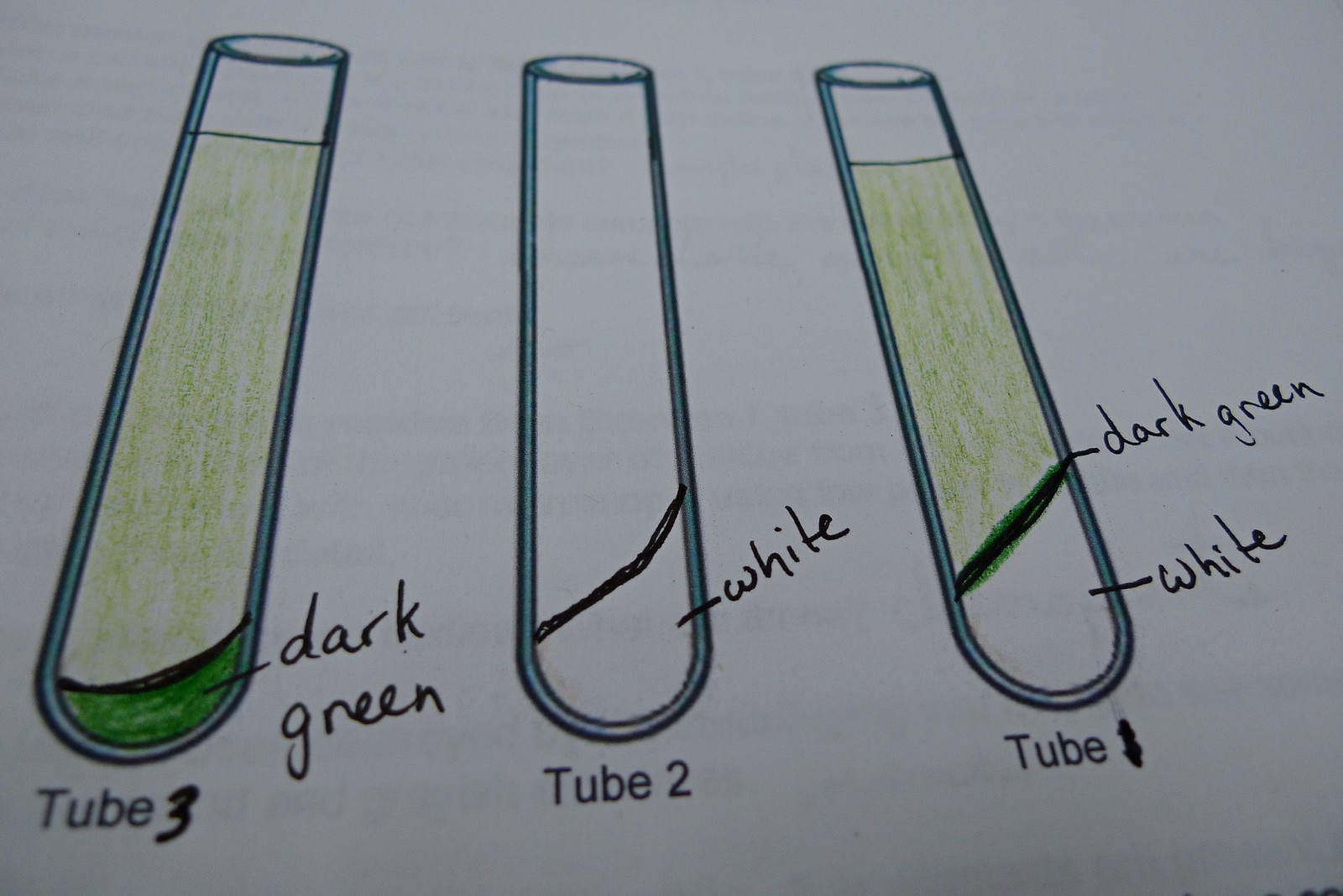The image is an illustration of three labeled test tubes on a plain white sheet of paper. The test tubes are arranged from left to right as tube 3, tube 2, and tube 1. Each tube is depicted with clear detailing of the substances inside them. 

Tube 3, on the left, is mostly filled with a light green liquid, with a smaller section at the bottom labeled "dark green." Tube 2, in the middle, shows a white substance at the bottom, with the label "white." Tube 1, on the right, is predominantly filled with a light green liquid, followed by a thinner band of dark green, and finally a section of white at the bottom. The illustration is clear and detailed, indicating layers of different colored substances, all against a plain white background.